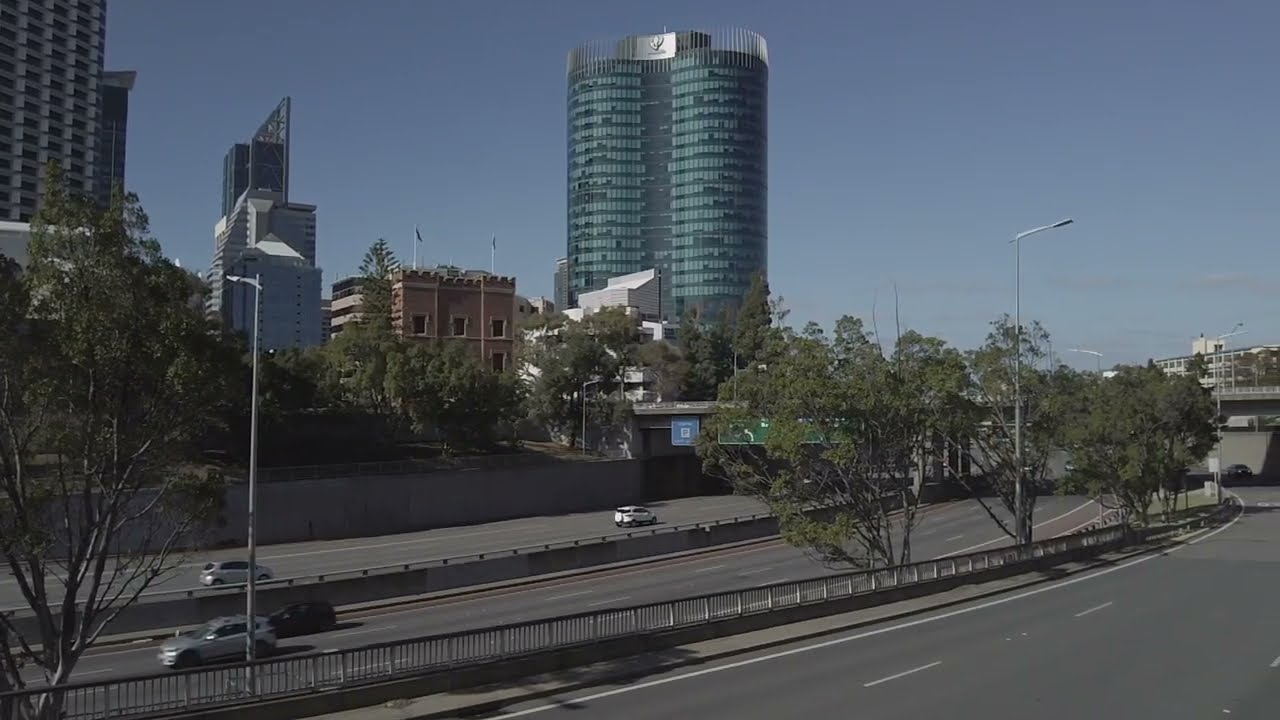This full-color photograph captures a bustling city scene taken outdoors during the daytime under a bright, mostly cloudless sky. The image spans a wide freeway with multiple lanes of traffic flowing in both directions, divided by medians populated with trees. A prominent feature is an overpass crossing the freeway, partially obscured by tree branches. On the right side of the photo, a striking tall building with a fancy architectural design stands out; it has a distinctive rounded shape and greenish glass windows, some with closed blinds. Adjacent to it, there is a smaller white building, followed by an older brick building, and other architecturally designed skyscrapers, one resembling a castle with flags flying on its roof. High above, billboards and street lamps dot the scene. The roadway dominates the bottom half of the photograph, while the upper portion showcases the city skyline, capped off by a clear blue sky with just a few faint clouds.